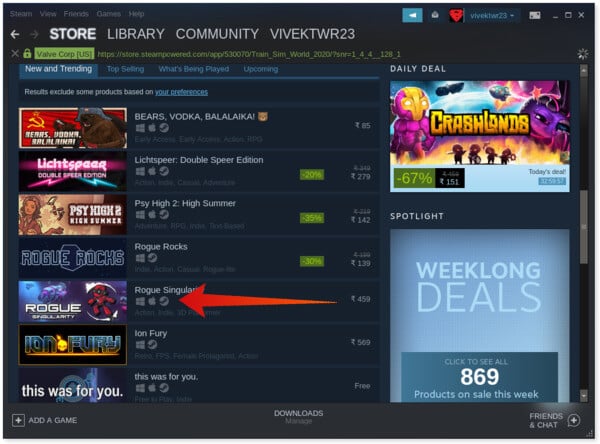The website displayed has a sleek black background with a navigation bar at the top. The bar includes sections titled: "Store," "Library," and "Community," alongside a user profile name accompanied by a number. The site is branded with the name "Value Corp."

Underneath the main navigation, the "Store" section is highlighted, showcasing the subcategory "New and Trending." This section consists of a comprehensive listing of available items complete with images. These items appear to be video game titles, with names like "Bears, Vodka, Baklava," "Lich," "Spear: Double Spear Edition," "Play High Two," "High Summer," "Rogue Rocks," "Rogue Singapore Singular," and "Iron Fury." A recommendation area labeled "This was for you" is also present.

On the right side of the page, there's a promotional image from a video game titled "Crash Crash Lands," featuring game characters. A green text indicates a 67% discount on this game. Below this, in light blue text, the section "Spotlight: Week-Long Deals" is displayed. There's also a darker box providing a link to view all "869 products on sale this week."

At the bottom of the website, a black bar runs across with options such as "Add a Game" on the left, "Downloads" in the center, and "Friends & Chat" on the right.